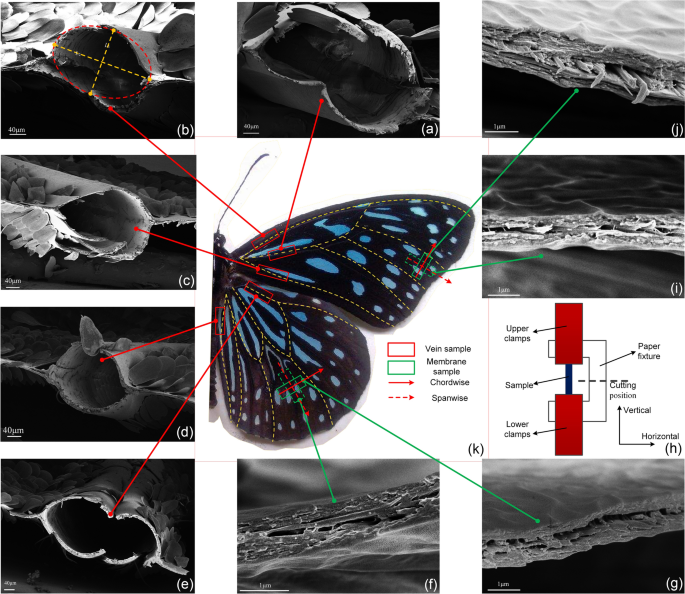The image depicts a detailed study of butterfly wing anatomy using a composite format. In the center is a colored close-up photo of a butterfly, showcasing its black wings adorned with blue specks. Surrounding this central image are black and white close-up photographs of various parts of the butterfly's wings, each placed in square boxes and labeled with letters A through G, I, and J; letter H is notably absent but is replaced by a detailed diagram in the form of a map depicting a part of the butterfly with a cylindrical element. Arrows connect each black and white photo to their corresponding location on the central butterfly's wings, providing a clear correlation between the parts and their positions. 

In the center, there's a key featuring a red triangle indicating vein samples and a green triangle for membrane samples. Additional detailed diagrams are included, highlighting intricate features such as the structure of veins and membranes, and explaining elements like upper clamps, paper fixture, cutting position, and lower clamps. This comprehensive setup not only names but thoroughly explains the different parts of the butterfly's wings, including samples and structural details, making it a highly informative visual guide.